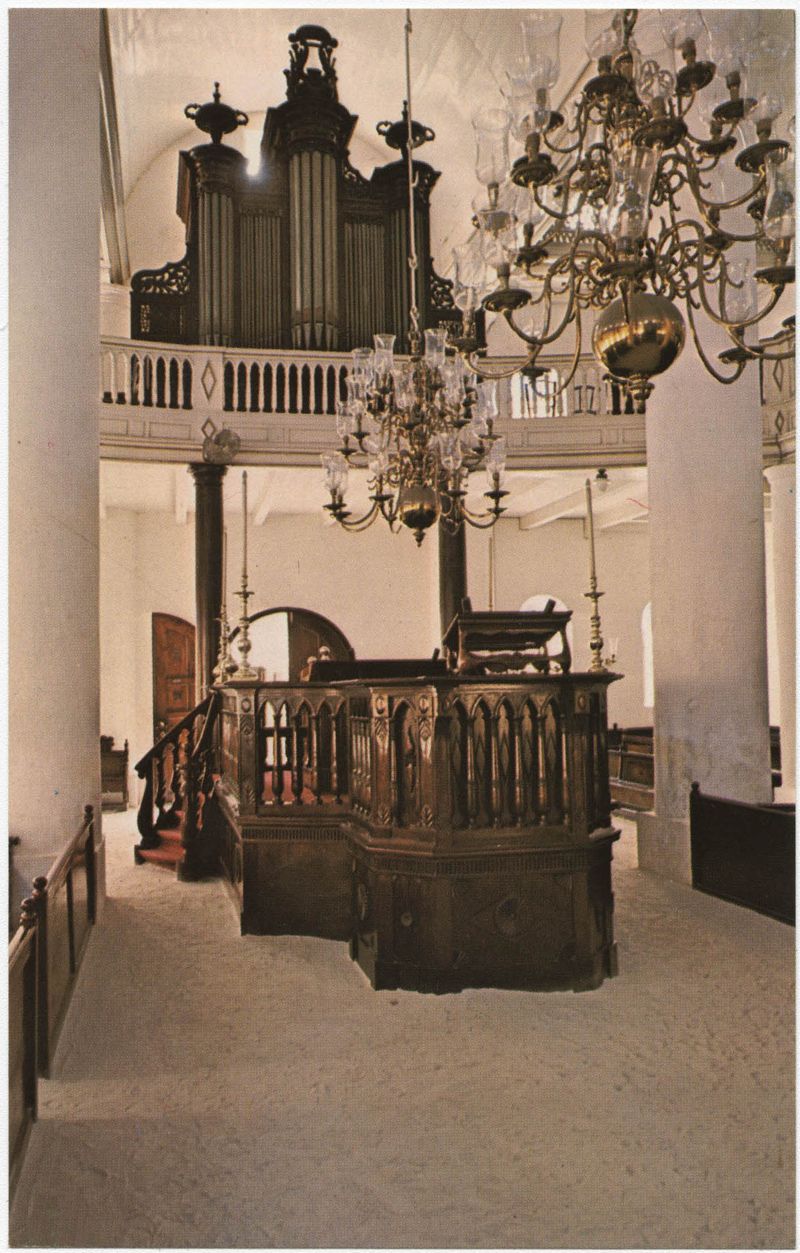This detailed color photograph, slightly grainy and taken in portrait mode, captures the ornate interior of a tall, solemn room, resembling a church. Dominated by hues of brown and cream, the scene features two elaborate brass chandeliers with gold details and many glass candle holders, hanging prominently in the foreground. The floor is beige, complementing the rich wooden elements throughout the room. Central to the composition is a grand wooden staircase, flanked by imposing marble pillars. The staircase leads to a second level featuring an intricate balcony with an elaborate sculpture above. This balcony is supported by three white columns on each side and enclosed by a white railing. At the front, there is a dark brown wooden dais or pulpit, suggestive of a platform for a speaker or potentially something musical. Adding to the architectural elegance is an oval opening at the back, framed by wooden doors, enhancing the room's sophisticated and ornate ambiance.